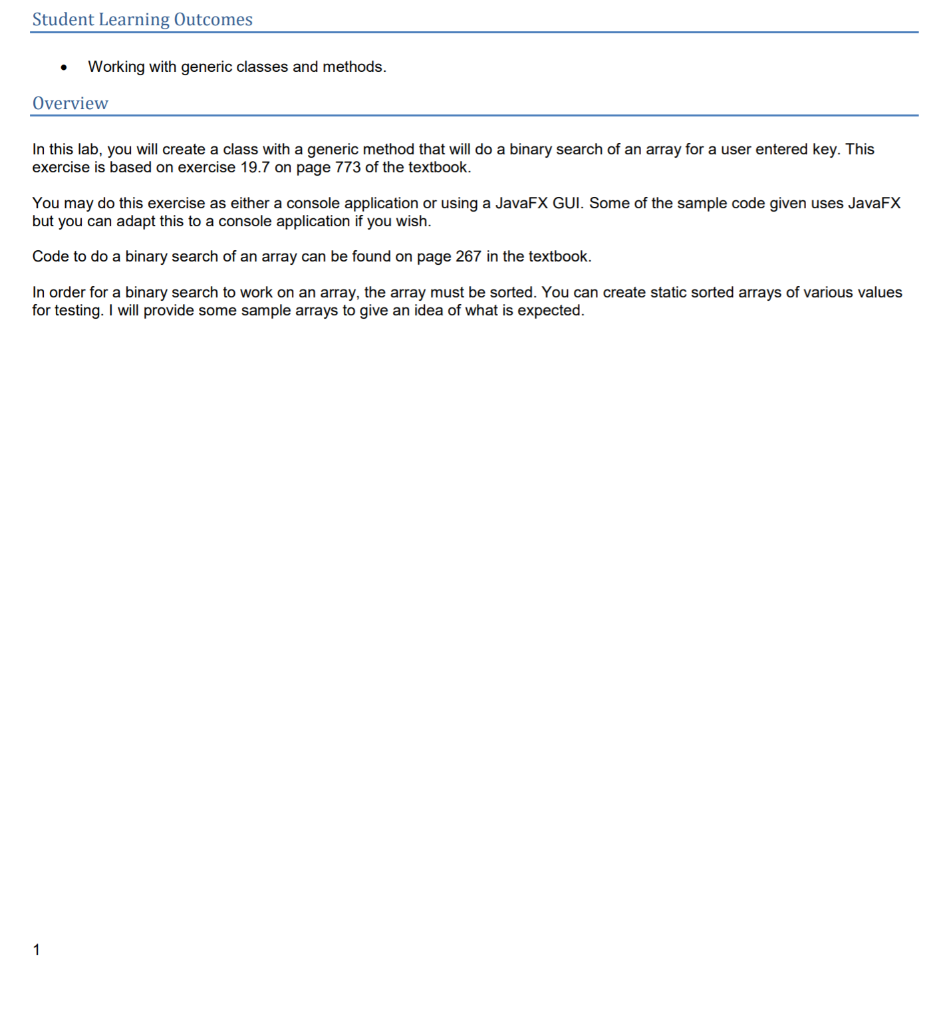The image features informative text and is formatted with specific sections and instructions. 

At the top left, the text "Student Learning Outcomes" is written in blue, with each word capitalized. Below this title is a blue horizontal line. The section begins with a black bullet point followed by the text in black font: "Working with Generic Classes and Methods."

Directly beneath this, the word "Overview" appears in blue, followed by another blue horizontal line. The main content consists of three paragraphs in black font:

- The first paragraph reads: "In this lab, you will create a class with a generic method that will perform a binary search of an array for a user-entered key. This exercise is based on exercise 19.7 on page 773 of the textbook."
- The second paragraph states: "You may complete this exercise as either a console application or using a JavaFX GUI. Some of the sample code provided uses JavaFX, but you can adapt it to a console application if you wish. Code for performing a binary search on an array can be found on page 267 of the textbook."
- The third paragraph explains: "For a binary search to work on an array, the array must be sorted. You can create static sorted arrays with various values for testing. I will provide some sample arrays to give an idea of what is expected."

This structured presentation offers a comprehensive overview of the task, specifying the resources and approaches one can use to complete the exercise.